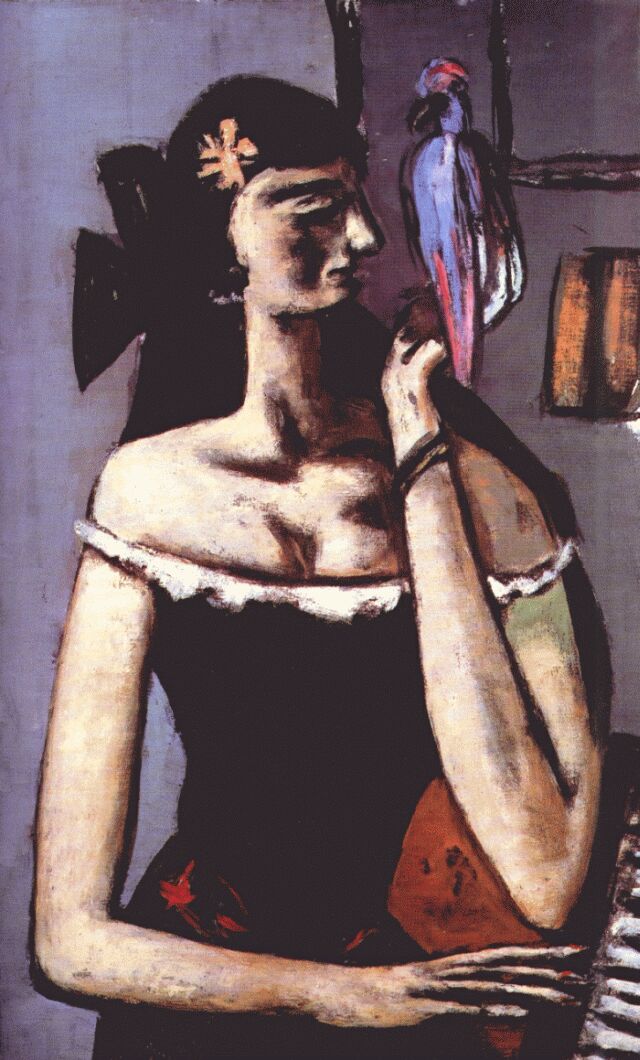This captivating painting, reminiscent of Picasso's 1920s cubist style, showcases a highly stylized woman with exaggerated features and vivid colors. The woman, depicted as tall and slender with dark, flowing hair, is wearing a black dress with a distinctive red belt draped across her shoulders. A striking pink flower adorns her hair, adding a touch of softness to her figure. 

Her posture is intriguing; she sits gracefully, her head turned to the right in profile, her eyes seemingly closed, perhaps lost in thought. Her right hand extends across her front to rest on a table or a piano, while her left hand, bent at the elbow, gently cradles a colorful parrot. This parrot, perched on her shoulder, is an eye-catching blend of purple and blue with red accents on its head and tail, and a bit of white at the edges of its wings.

The background features stark contrasts, with a plain wall on the left adorned only with two mysterious black triangles. On the right, a more detailed backdrop includes an orange bookshelf or a lampshade, adding depth to the scene. Overall, this intricate composition invites viewers to ponder its myriad of details and the emotions it evokes.